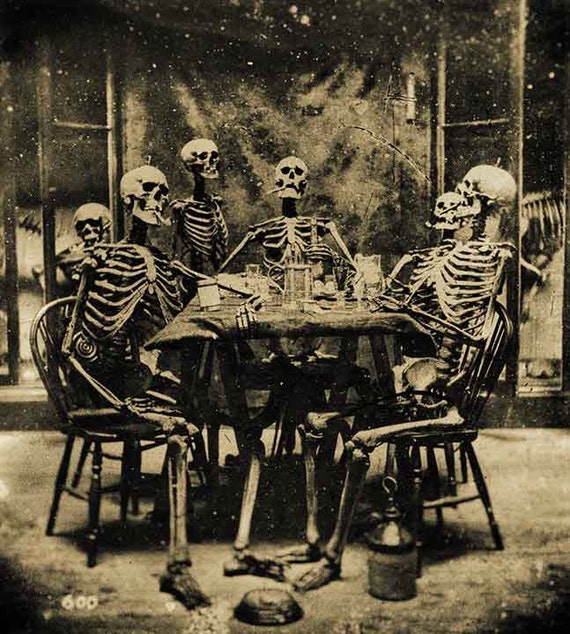An aged, sepia-toned image presents a macabre scene of six skeletons arranged around a worn wooden table, seemingly engaged in a lifelike gathering as though they were still alive. The table, draped in a cloth, is cluttered with glassware and other objects, evoking the sense that these skeletons might be in the midst of a poker game or perhaps enjoying a drink. Some skeletons have cigarettes or pipes in their mouths, underscoring a possible anti-smoking message. Two of the skeletons are standing while the others are seated, their bony elbows perched nonchalantly on the table. In the background, a dark, dreary room reminiscent of the Addams Family's abode features what may be wooden supports, possibly framing a window or a glass door. Additionally, a lantern rests on the floor near one of the chairs, and a bell shape can be discerned nearby. The lower left-hand corner of the image bears the cryptic number "600600" in white. Overall, the scene's limited color palette, dominated by black and sepia tones, enhances its eerie, antiquated atmosphere.